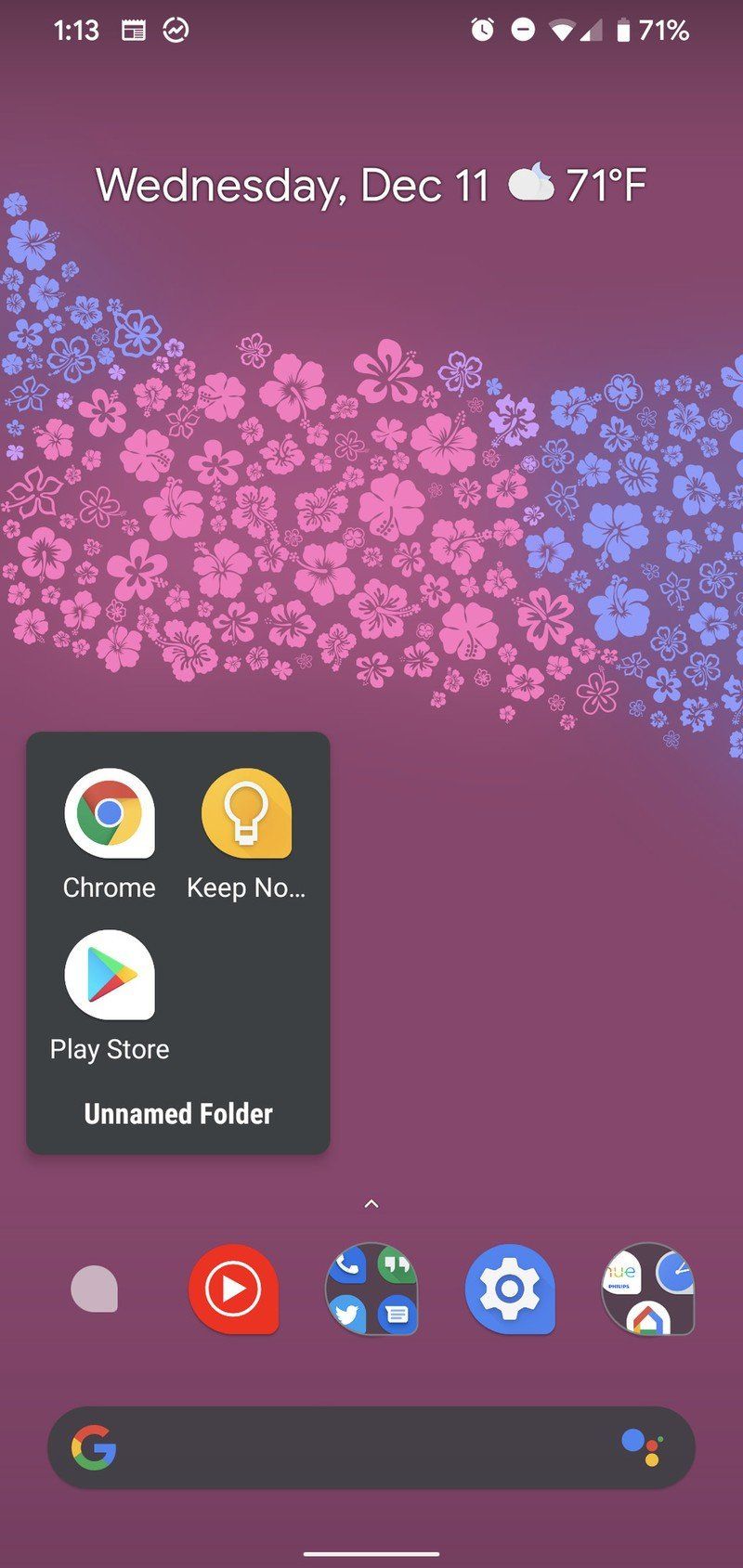The screenshot from the phone displays several elements detailed below:

- **Time and Status Indicators**: The time displayed is 1:13, and the battery level is at 71% with a signal strength of 2 out of 5 bars. Icons for an alarm clock and timer are also visible.

- **Date and Weather Information**: Beneath the time and status indicators, the screen shows the date as Wednesday, December 11th. The weather is indicated as 71°F with a cloudy icon.

- **Background Design**: The background features a purple hue adorned with blue flowers on the left and right sides, and pink flowers in the middle, arranged in a striped pattern.

- **App Icons and Labels**: 
  - A black box at the bottom contains several app icons:
    - A Chrome icon, labeled "Chrome".
    - An orange circle with a flash icon and a light bulb, partially labeled "Keep NO...".
    - A Google Play icon, labeled "Play Store".
    - An unnamed folder, presumably containing other applications.
    - A red circle with a play button icon.
    - A blue circle with a gear symbol.

- **Google Search Bar**: A black bar at the bottom features the Google logo, presumably for initiating a Google search.

This detailed description offers a comprehensive overview of the phone screenshot, covering all visible elements and their arrangement.